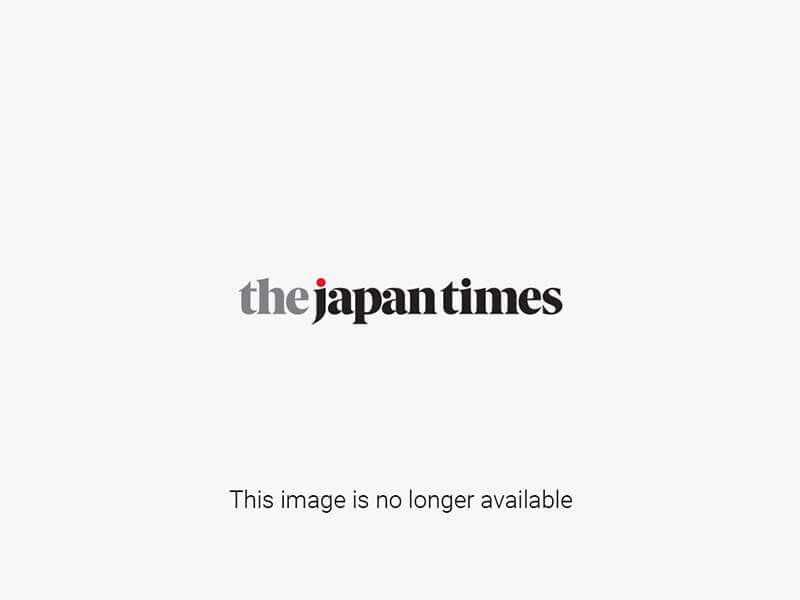The image features four young Asian individuals, likely in their late teens or twenties, standing in what appears to be a photo shoot or team presentation. From left to right, there are two boys with short dark hair and two girls with longer dark hair, all dressed identically in white down jackets adorned with various advertisements including prominent logos such as Visa, Phoenix, and Snow Japan. They are also all wearing red long pants. Each person has their right arm extended towards the center, touching their forehands together, and they are all smiling. The backdrop consists of a repeating pattern of squares, alternating between “Snow Japan” in red letters and an illustration of the Japanese flag—with the letters S-A-J beneath the red circle. The overall impression suggests they may be part of a sports team or promotional team related to snow sports or a related event in Japan.